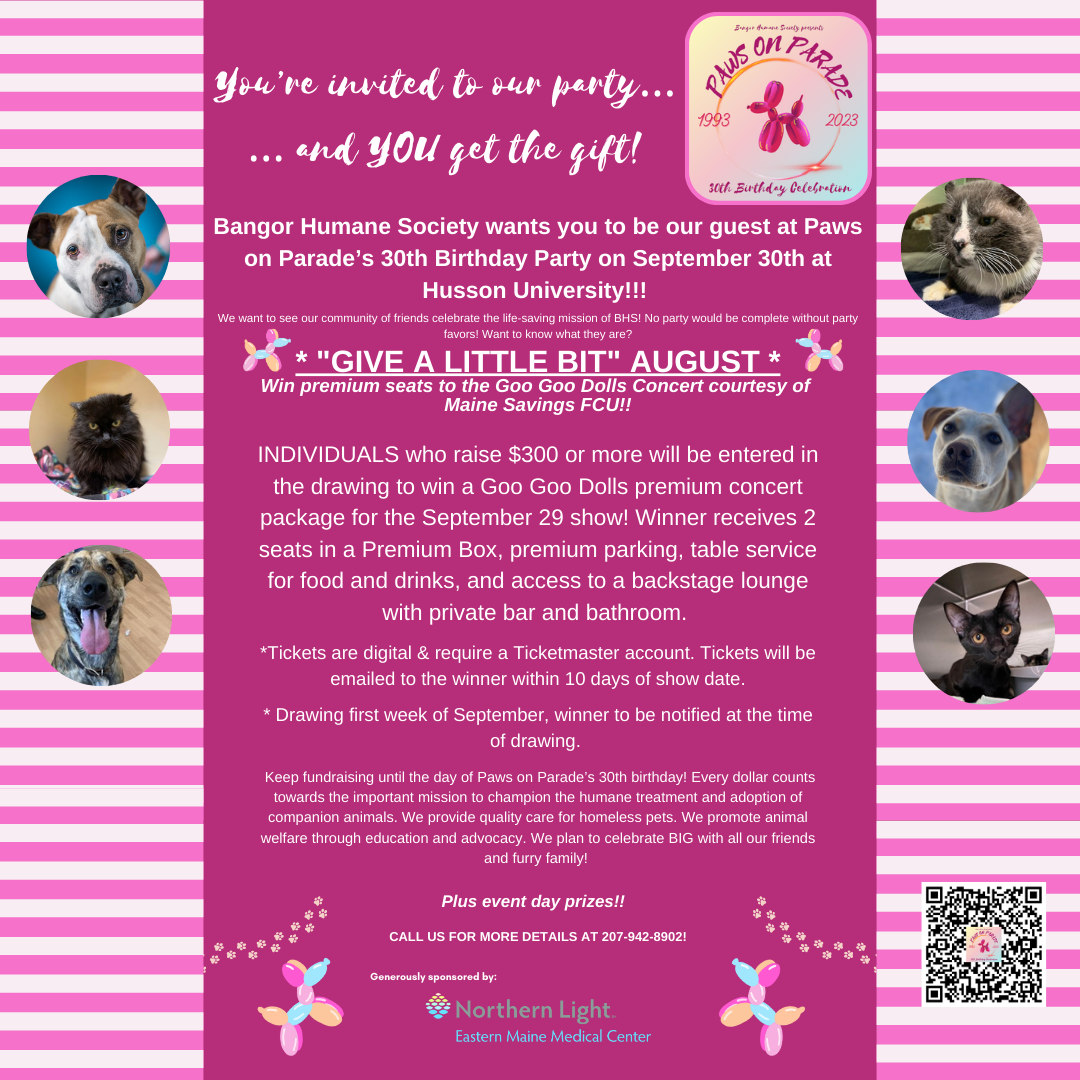This advertising poster features a vibrant design in shades of pink and white. The background displays alternating vertical bars of light and dark pink on both the left and right sides. On the left, three round icons are arranged vertically: a brown and white dog at the top, a black cat in the middle, and another brown dog with a brown background at the bottom. The right side mirrors this arrangement with a gray and white cat at the top, a white dog with brown ears in the middle, and a gray kitten at the bottom. 

The central section of the poster features a vivid dark pink background with bold white text that reads: "You're invited to our party and you get the gift." Positioned to the right is a square icon that says "Paws on Parade" with a balloon dog in the center, marked "1993" on the left side and "2023" on the right, celebrating the "30th Birthday Celebration."

Below this, in bold white lettering, it announces: "Bangor Humane Society wants you to be our guest at Paws on Parade's 30th birthday party on September 30th at Husson University." Flanking this title are two colorful balloon animals, one on the left and one on the right.

Further down, there is a title that reads "Give a Little Bit" followed by an opportunity to "Win premium seats to the Goo Goo Dolls concert courtesy of Maine Savings FCU," along with details about event activities including a show, refreshments, raffles, and event day prizes. The text suggests contacting for more details and provides a phone number.

At the very bottom, two more balloon animals frame the text "Northern Light Eastern Maine Medical Center," presented in a multi-hue gradient lettering.